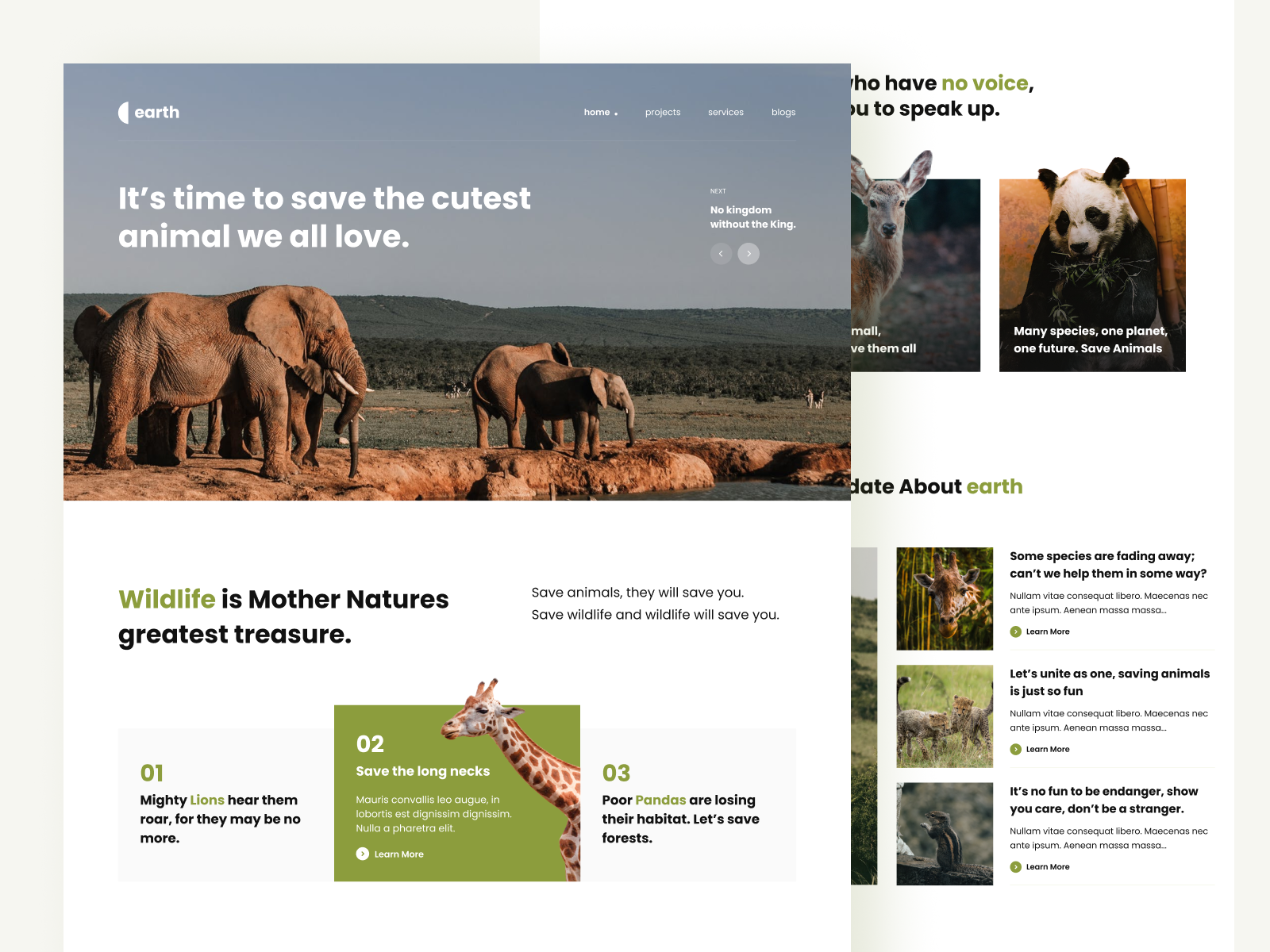Here is a more detailed and cleaned-up caption for the image described:

---

A visually appealing website with off-white borders on the left side and a partially white top section features a striking image of elephants standing on a brown rocky surface near water. The background includes lush grass, trees, rolling hills, and a clear blue sky, enhancing the natural beauty of the scene. In the top left corner of the sky in the image, text reads, "Earth: It's time to save the cutest animal we all love".

Below this main image, on a white background, a bold heading declares, "Wildlife as Mother Nature's Greatest Treasures". The content is segmented into sections:

1. "01: Mighty lions hear them roar, for they may be no more", accompanied by an image of a majestic lion.
2. "02: Oh, to save the longnecks", featuring a giraffe facing towards the left.
3. "03: Poor pandas losing their habitats", accompanied by an image of a panda.

In the upper right corner of the webpage, there are additional smaller images of a deer and a panda. However, some text is cut off by the main picture of the elephants below.

Further down, more animal images are displayed, including a giraffe, cheetah cubs, and a chipmunk. Adjacent to each image, there is informative black text along with a 'Learn More' button, inviting users to explore further details about these animals.

---

This caption provides a seamless, descriptive overview of the elements displayed on the website while encapsulating the essence and purpose of the content presented.